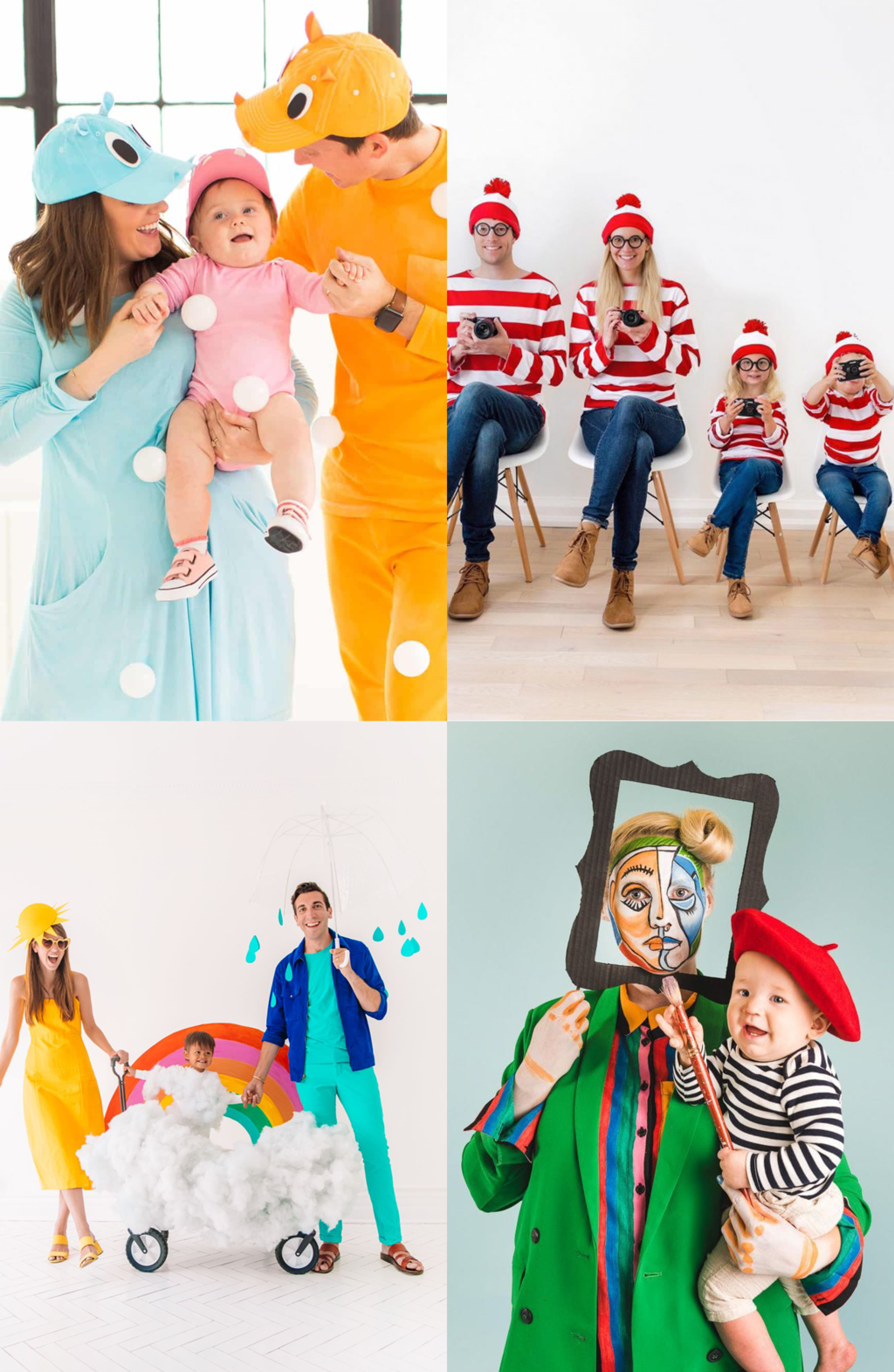This collection of four family photographs features various creative costume themes. The upper left image showcases a family of three with a fun, cartoonish theme: the mother has long brown hair and wears a light blue costume and a hat with eyes, the father is in a similar outfit but in a yellowish-orange color, and their smiling baby is dressed in a similar pink outfit. In the upper right photo, a family of four is dressed as "Where's Waldo" characters, wearing white and red striped hats and sweaters, blue jeans, and brown sneakers, sitting on wooden stools against a white background and possibly holding cameras. The bottom left image depicts a couple and their baby; the woman is dressed in a bright yellow dress and hat, while the man wears light blue pants and a shirt, holding an umbrella under rainy scenery. The baby is dressed as a cloud on wheels with a vibrant rainbow behind it. In the bottom right photo, a woman is dressed as a Picasso painting, wearing a green painting smock and holding an empty frame in front of her face, which is painted in a Picasso style. The baby, dressed in khakis, a black and white striped shirt, and a red beret, holds a paintbrush. There is no visible text in any of the photos.